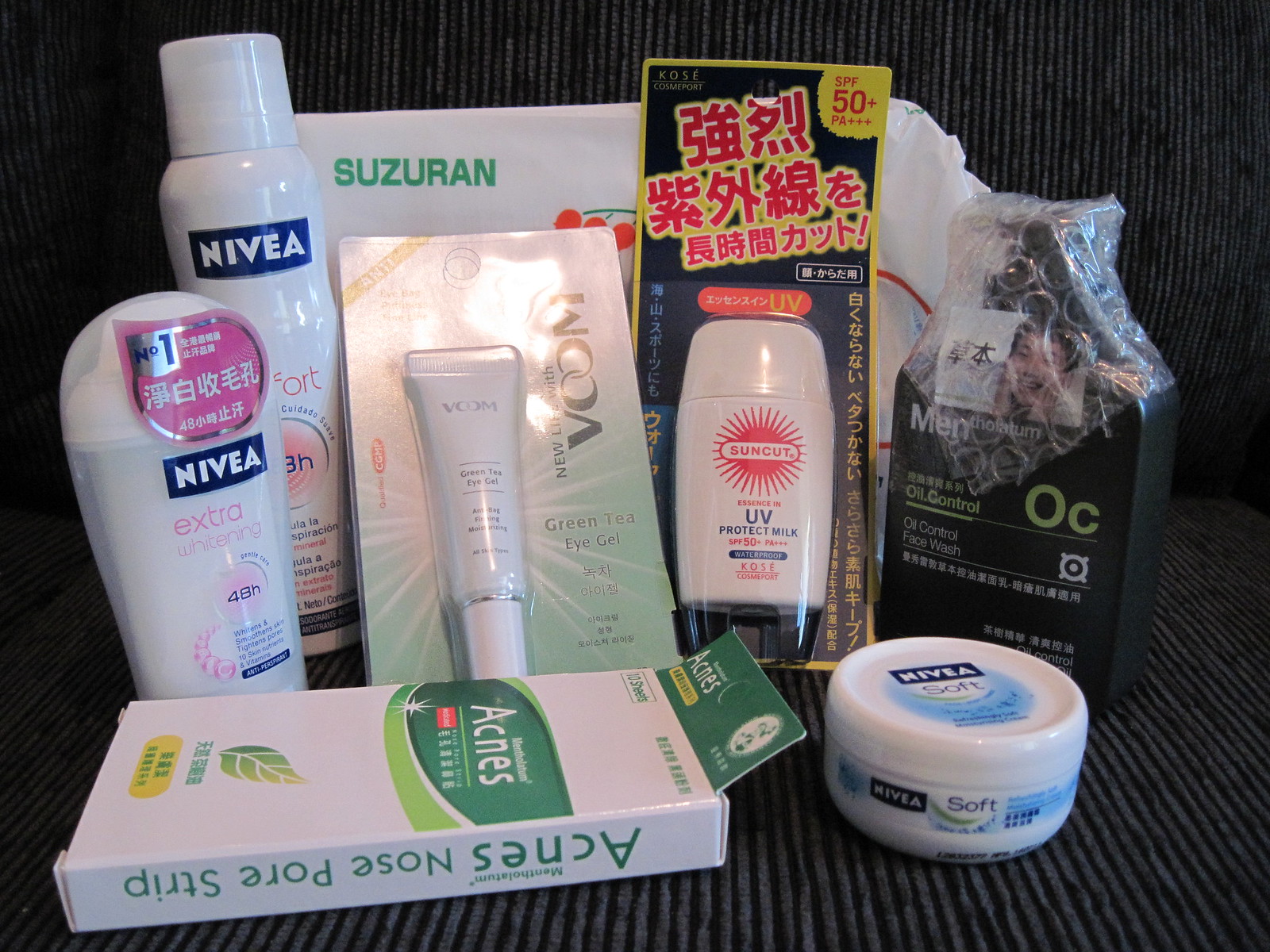In the photograph, a variety of toiletries are arranged against a black, textured background that resembles corrugated cardboard or velvet. The setup appears to be leaning against a 90-degree angled surface, creating a sophisticated, cohesive aesthetic. From left to right, the items include:

- A deodorant stick
- A body spray or possibly a spray deodorant

Leaning against the background is a product labeled "Suzuran" in green text, though its exact nature is unclear. In front of Suzuran, several smaller items are positioned:

- An eye gel
- UV protect milk, featuring text in an Asian language on the package
- An oil control face wash marked with the word "Men" and initials "O.C." in light green lettering

On the lower part of the arrangement:

- A box of nose pore strips, labeled in green on a white background
- A jar of Nivea Soft cream in white and blue

Each item is meticulously placed to create an organized and visually appealing display against the uniform dark background.